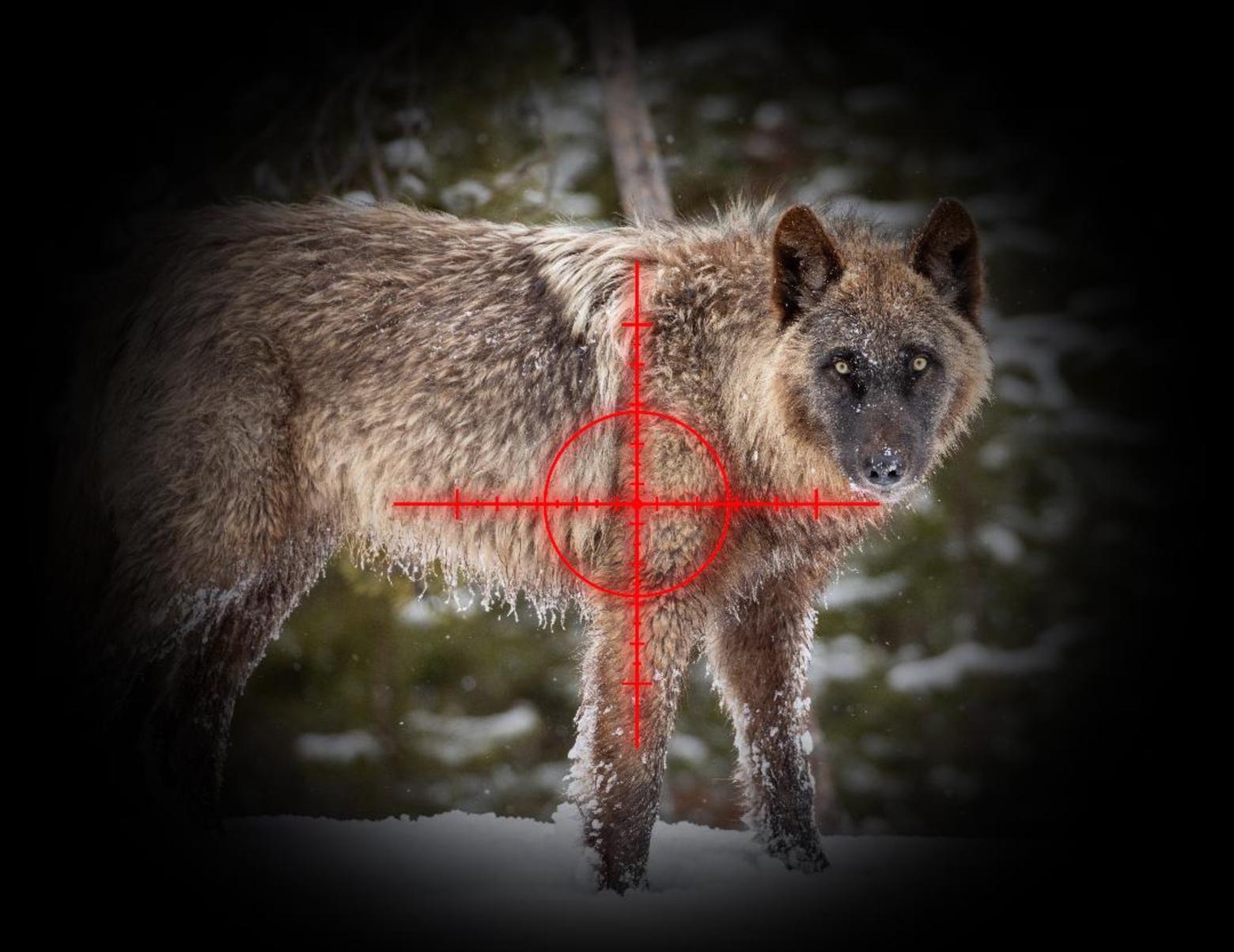The image features a brown-furred wolf with a distinctive black face, standing alert on a snowy terrain with shiny, vivid green leaves and snow-covered trees in the background, suggesting a winter setting. The wolf's head is turned to its right, gazing directly at the viewer with bright, light yellow eyes. Superimposed over the image is a red crosshair target, consisting of a circular outline with a dot in the center and a cross running through it, indicating a hunting scenario. The photo also has a black vignette effect around the edges, adding a dramatic focus on the animal. The wolf's ears are pointy, and its wet nose glistens, highlighting its attentive stance. The background is slightly blurred, emphasizing the wolf and the crosshair as the central elements of the scene.